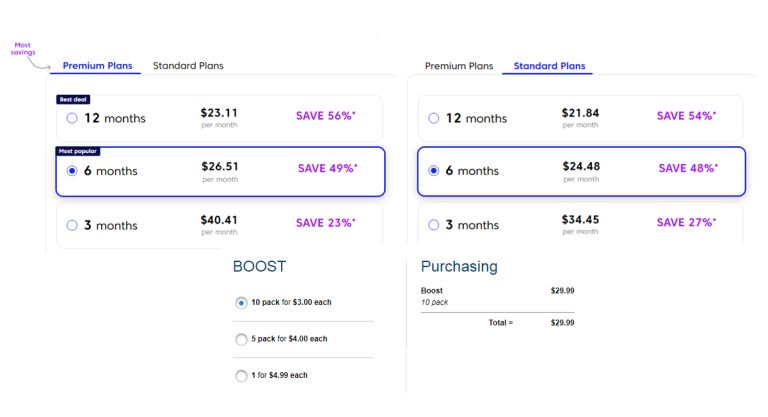The image depicts an online shop website offering various subscription plans. The layout is divided into two sections: the left and the right. 

### Left Section
At the top of the left section, the heading "Premium Plans" is displayed in blue text. Below it, "Standard Plans" is listed in a smaller font. This section further breaks down into detailed rows of options:

1. **First Row ("Best Deal")**
   - A circle (currently unchecked)
   - **Duration:** 12 months
   - **Price:** $23.11 per month
   - **Savings:** 56%, highlighted in purple text

2. **Second Row**
   - A circle (currently checked)
   - **Duration:** 6 months
   - **Price:** $26.51 per month
   - **Savings:** 49%, with an asterisk, highlighted in purple text

3. **Third Row**
   - A circle (currently unchecked)
   - **Duration:** 3 months
   - **Price:** $40.41 per month
   - **Savings:** 23%, highlighted in purple text

4. **Additional Options**
   - **Boost Packs:** 
     - **10 Packs for $3 each** (circle checked)
     - **5 Packs for $4 each** (circle unchecked)
     - **1 Pack for $4.99 each** (circle unchecked)

### Right Section
This section has headings for both "Premium Plans" and "Standard Plans." The "Standard Plans" option is highlighted in blue, while the "Premium Plans" option is in black text. The options are detailed in three rows:

1. **First Row**
   - A circle (currently unchecked)
   - **Duration:** 12 months
   - **Price:** $21.84 per month
   - **Savings:** 51%

2. **Second Row**
   - A circle (currently checked)
   - **Duration:** 6 months
   - **Price:** $24.48 per month
   - **Savings:** 48%

3. **Third Row**
   - A circle (currently unchecked)
   - **Duration:** 3 months
   - **Price:** $34.45 per month
   - **Savings:** 27%

### Purchase Summary
- **Boost Packs:**
  - **10 Packs**: Priced at $29.99
- **Total Pricing**: $29.99

The website provides a comprehensive breakdown of premium and standard subscription plans, including the duration, monthly cost, and percentage savings. It also highlights special offers and additional boost packs with various pricing options.